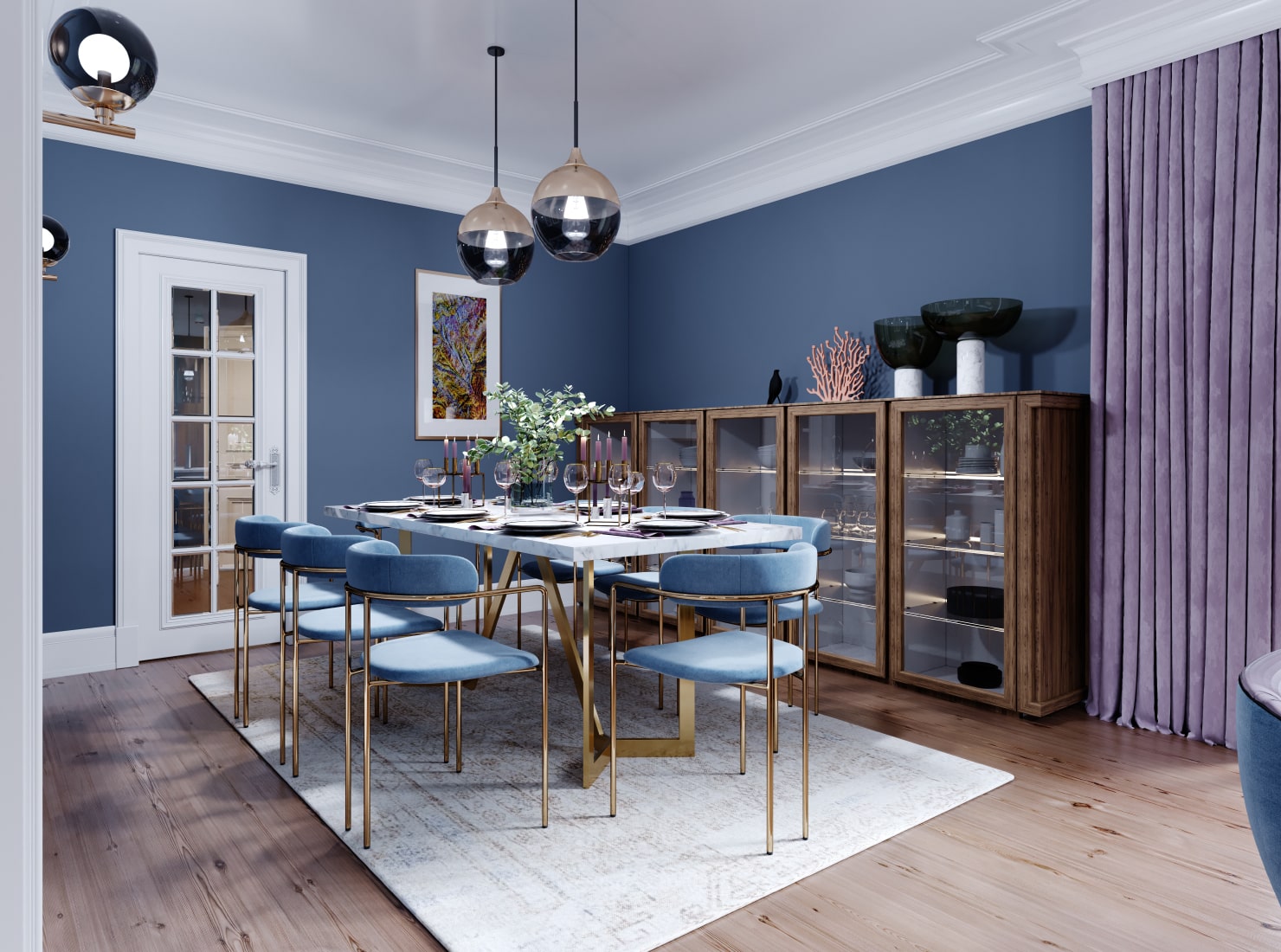This photograph captures the interior of a stylish dining room adorned with postmodern design elements. The room features cornflower blue walls contrasted by a white ceiling and light wood flooring partially covered by a white rug. The central piece is a marble-top dining table, fully set with plates, glasses, and candles, with a plant as the centerpiece. Surrounding the table are sleek, modern blue chairs with metallic legs.

Above the table hang two striking orb-shaped light fixtures, illuminating the entire setup. Along the back wall, a glass display case or China cabinet showcases silverware, dishes, and bowls, topped with a coral decoration and a bird figurine. Pale purple curtains add a soft touch to the room's ambiance. Additionally, there is a door with see-through metal panes providing a view into an adjacent room, and a painting on the wall that adds an artistic flair to the space.